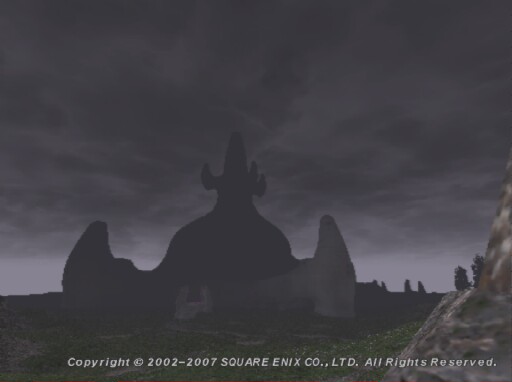Caption:  
A dark, atmospheric screen capture depicts an animated scene, possibly from a video game. The image showcases a unique, desert-like cactus-shaped building under a stormy, grey sky. The foreground is dotted with rocks, and the overall color palette consists of varying shades of grey and black, which obscure finer details. The screenshot is marked with a copyright notice, "2002-2007 Square Enix Company Ltd. All rights reserved," indicating that it could be an official image from a game or an animated scene.